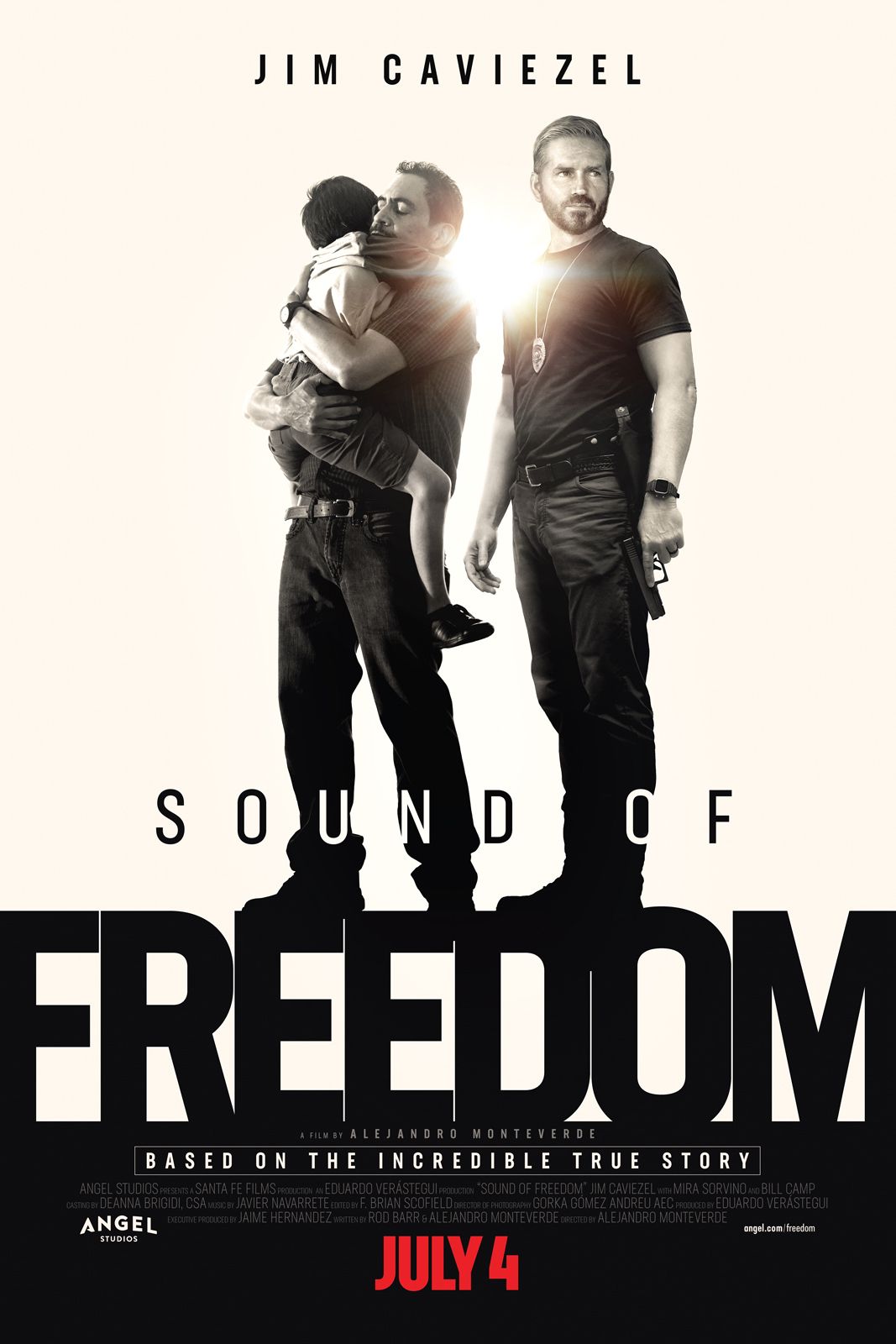The movie poster for "The Sound of Freedom" prominently features the actor Jim Caviezel at the top. The background is a tan, off-white color, and the centerpiece of the poster is two men depicted in black and white. They are dressed in dark t-shirts, dark pants, and boots, suggesting they are either policemen or military personnel. The man on the right wears a badge around his neck on a chain and holds a pistol. The man next to him appears to be Hispanic and is cradling a small child whose face is not visible but is wearing shorts. Rays of sunlight emerge between the two men, creating a dramatic effect.

The title "The Sound of Freedom" is prominently displayed in black letters, with "FREEDOM" in large, bold capital letters at the bottom, giving the impression that the men are standing on it. Just above "FREEDOM," a black banner reads "Based on the Incredible True Story" in white letters, and below it, "July 4" is highlighted in large, bold red letters. Additional text at the bottom credits the film's director, Alejandro Monteverde, alongside writers Rob Barr and Alejandro Monteverde, and producer Jamie Hernandez. The film, produced by Angel Studios, also stars Mira Sorvino and Bill Camp, and is based on the true story of a man who rescues children from child predators. A website, angel.com/freedom, provides more information about the film.